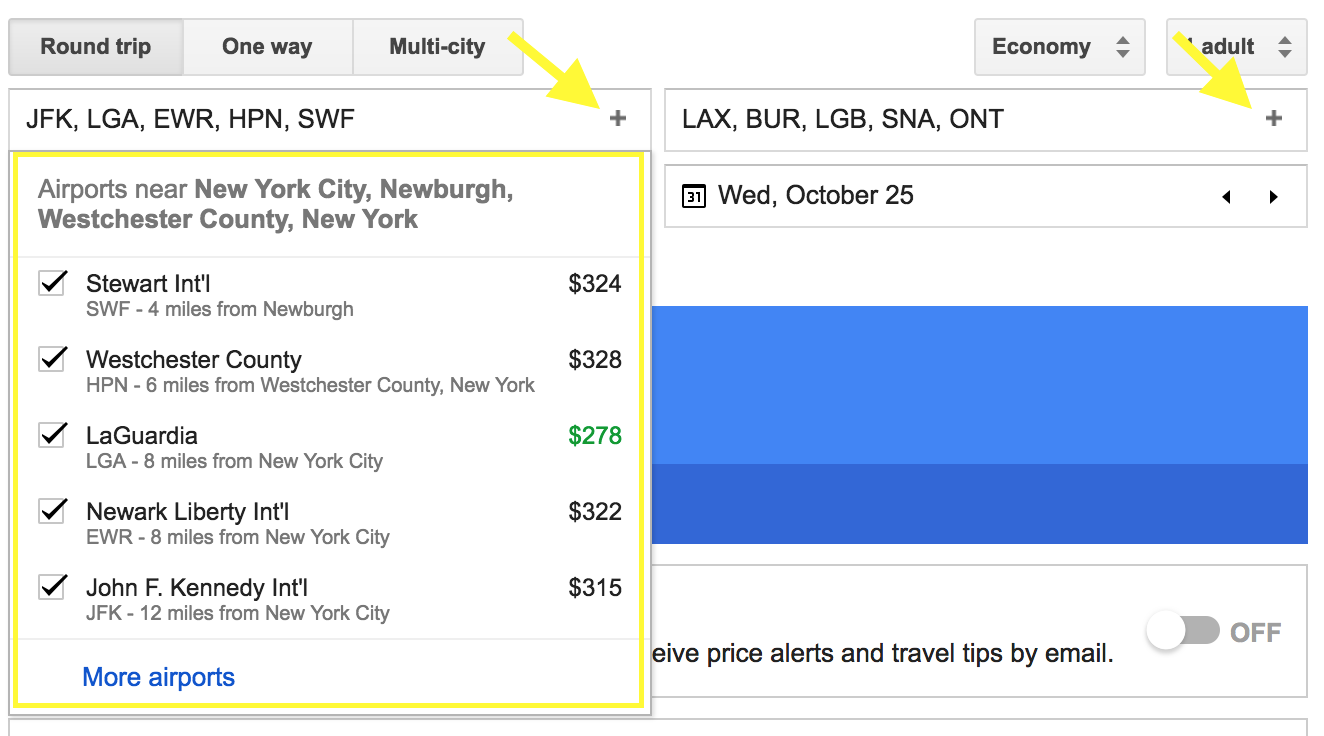This is a cropped screenshot from a flight selection page on a travel website, meticulously detailing various elements of the interface. At the top left corner, there are three distinct tabs labeled "Round-trip," "One-way," and "Multi-city," providing different flight itinerary options. 

On the left side, two dropdown menus are visible. The first box contains the option "Economy," while the second box indicates "Adult." Each of these boxes has an arrow pointing up and another pointing down to adjust the selections accordingly.

Directly below these dropdown menus is a larger input box. At its top, airport codes are displayed in abbreviated form, and to the right, there's a prominent plus sign. An added yellow arrow points at this plus sign, indicating its function to add more departure airports.

On the right side, two horizontal input boxes align sequentially. The top box lists airport codes for the return flight, distinguishably different from the departure ones. Beside it, another plus sign allows adding additional return airports. Yellow arrows point at both plus signs, clearly marking areas to modify departure and return airport selections.

Further down, a box displays the selected date, "Wednesday, October 25th," flanked by left and right arrows for adjusting the travel date.